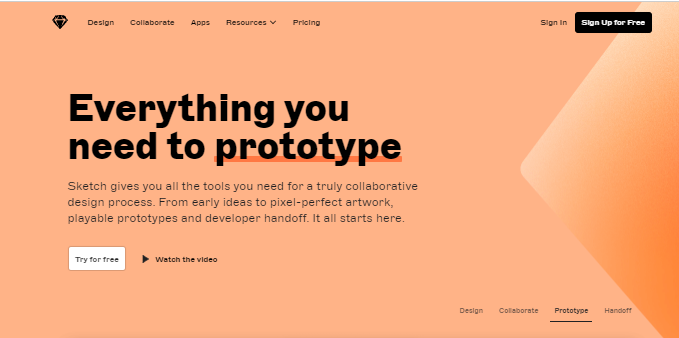The webpage features a design with a pale peach background on the left-hand side, transitioning to an ombre effect triangle on the right that shifts from orange to pale orange or peach. At the top, there's a black diamond symbol followed by a navigation menu with the titles: Design, Collaborate, Apps, Resources, and Pricing. In the upper right-hand corner, there are options to Sign In and a prominent Call to Action button labeled "Sign Up for Free" in white text on a black background.

The main headline, in large, bold black letters, states: "Everything you need to prototype," with the word "Prototype" underlined in orange. Below, a descriptive paragraph reads: "Sketch gives you all the tools you need for a truly collaborative design process from early ideas to pixel-perfect artwork, playable prototypes and developer handoff. It all starts here." Beneath this text lies another Call to Action button with the text "Try for Free" in white, followed by a black right-facing triangle and the option to "Watch the Video."

In the lower right-hand corner, there are words summing up the process: Design, Collaborate, Prototype, and Handoff, where "Prototype" is underlined in black.